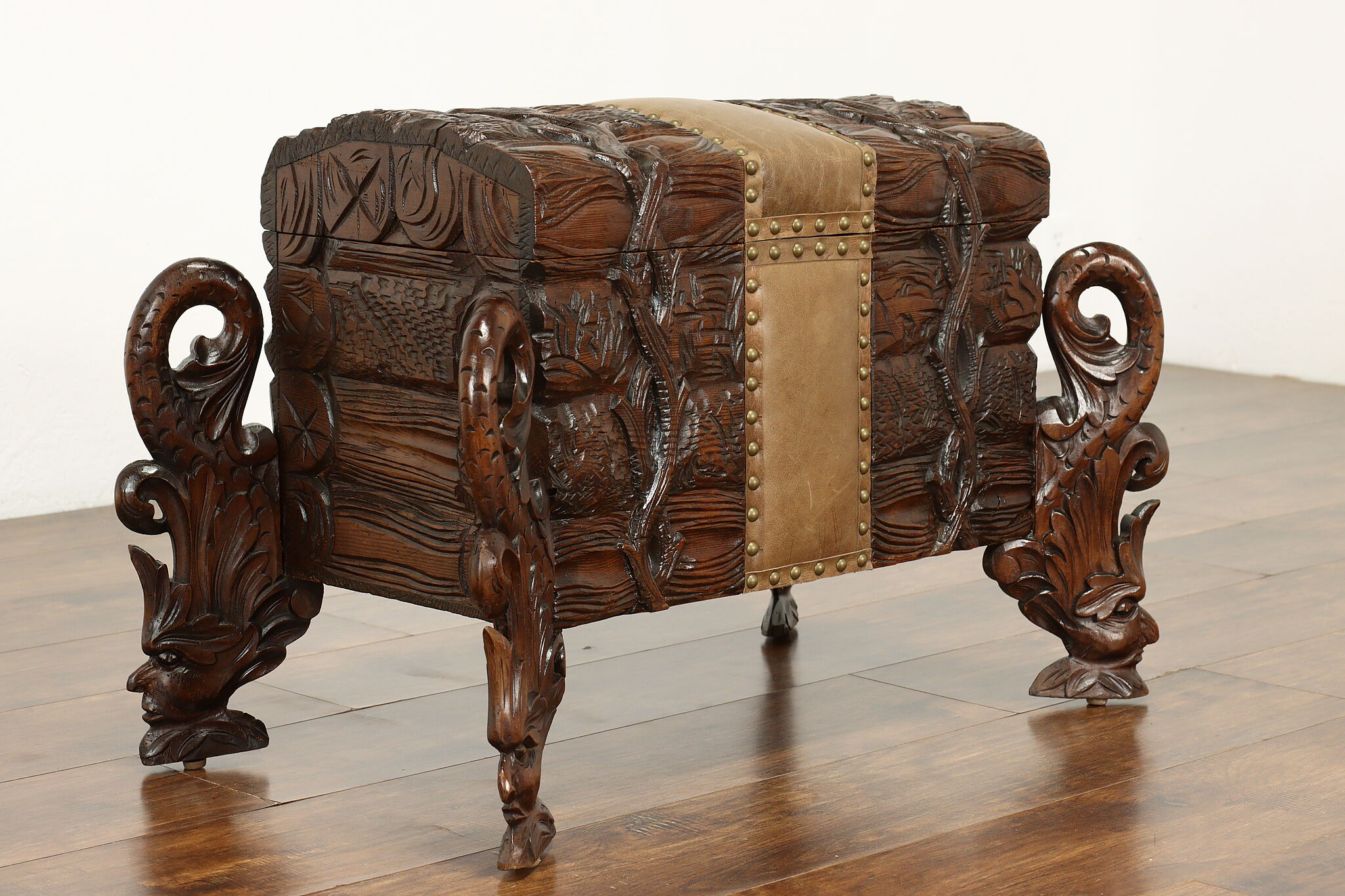This is a high-resolution, landscape-format photograph of a very elaborate and ornately carved wooden chest, displayed against a white background with rich brown wood flooring. The chest, made from a deep, rich mahogany wood, exhibits an old-fashioned aesthetic with intricate details. It stands on four curvy legs, each adorned with carvings that resemble faces, feathers, fish scales, and tails, contributing to an overall fantastical motif. The legs, evocative of vines and leaves, lift the chest about 8-10 inches above the ground. The center of the chest features a tan leather band, studded with medium-sized brass-like studs, adding to its ornate appearance. Additionally, a metallic gold strip, around 3-4 inches wide, runs horizontally across the lid and extends down the sides, enhancing the chest's opulent look. The lid is closed, seamlessly integrated into the chest's intricate design, making the opening mechanism inconspicuous. The wood appears varnished, contributing to its shiny and expensive look.